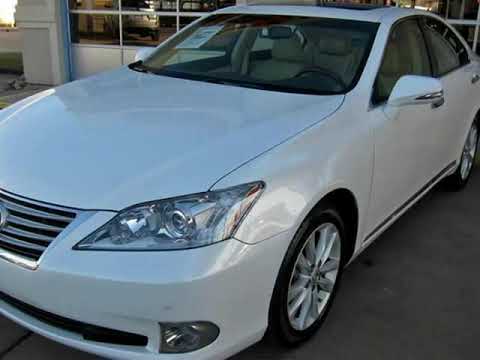The image features a pristine white sedan, prominently occupying the frame, with a slight shadow cast upon it. Captured from an angled front-left perspective, the photograph reveals the entirety of the car's hood, most of the front, including the left headlights, grill, and both the front and back tires on the driver's side. The front tire is black with a silver hubcap featuring slots and visible lug nuts. The car's body has a distinctive black strip running along the bottom edge of the doors from the front to the back tires, and the side mirror, reflecting light, appears quite silver.

The windshield offers a glimpse of the interior, showing tan-colored seats with headrests. The headlight in the lower-left corner is shiny and translucent, while the grill beneath it is detailed with four silver lines and a scoop opening near the bottom. Adjacent to this is another light in the very bottom corner of the car’s front.

The vehicle is positioned on a dark gray surface, possibly asphalt, suggesting it is outdoors. The background includes a building with multiple square-patterned window panes, consistent with a garage or auto repair shop. The image captures a sense of cleanliness and newness, suggesting the car has been recently washed. The photograph itself is relatively square, providing a comprehensive yet detailed view of this well-maintained vehicle.